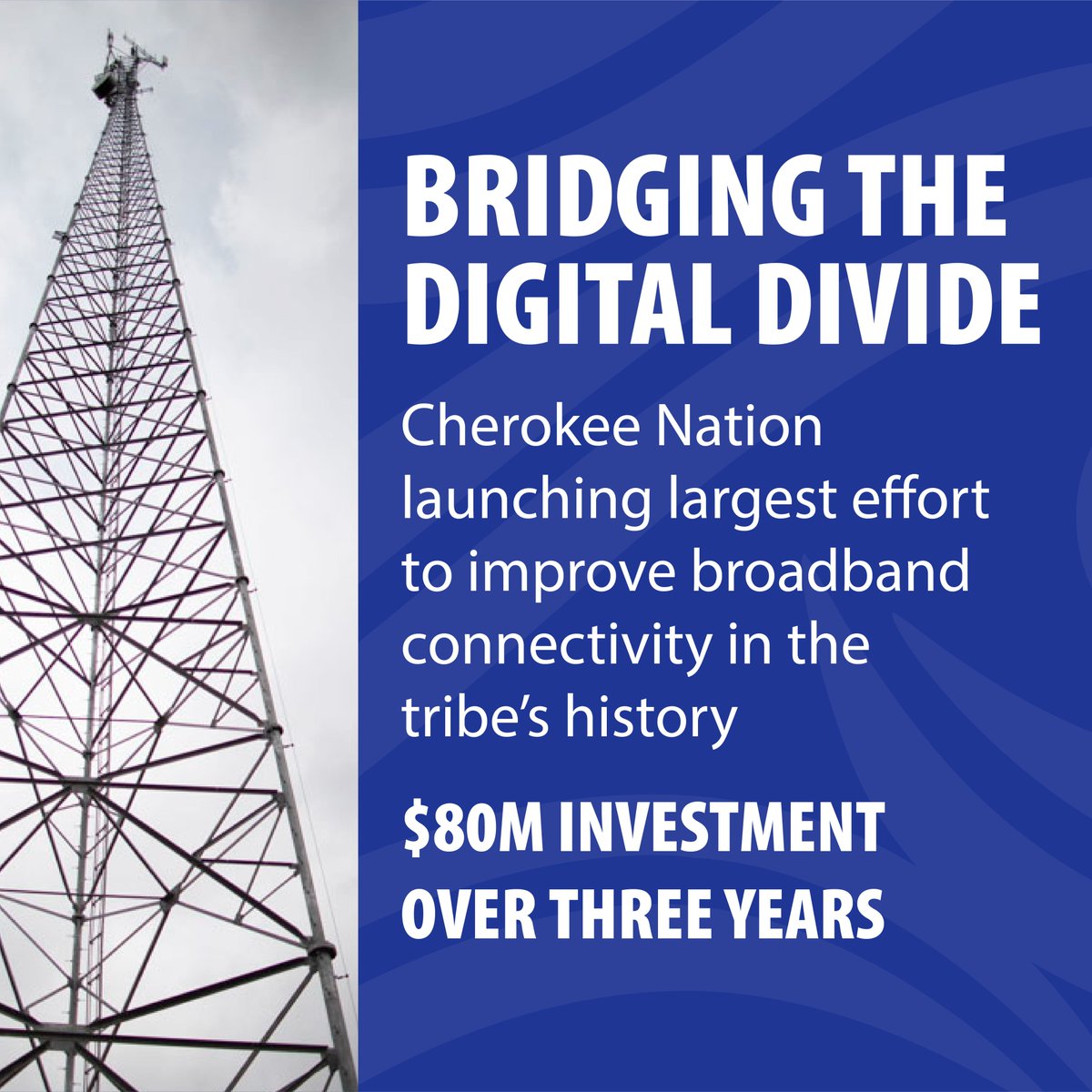The promotional flyer features a striking juxtaposition of imagery and text. The left one-third of the flyer is dedicated to a photograph of a triangular-shaped cell phone tower constructed from a metallic framework, standing tall against a gray sky backdrop. This tower, characterized by its three-sided structure, hosts a number of wires running down its center, with satellite dishes and antennas perched at the very top.

The remaining two-thirds of the flyer showcases a vibrant blue background adorned with lighter blue swirl patterns. Dominating the upper portion of this section, in bold, white capital letters, is the headline: "BRIDGING THE DIGITAL DIVIDE." This is followed by a significant announcement in white text, reading: "Cherokee Nation launches greatest effort to improve broadband connectivity in the tribe's history." 

Emphasizing the monumental nature of this initiative, the text concludes with a larger, bolded message stating, "$80 million investment over three years." The elements of the flyer collectively underscore a historic and substantial technological advancement for the Cherokee Nation.